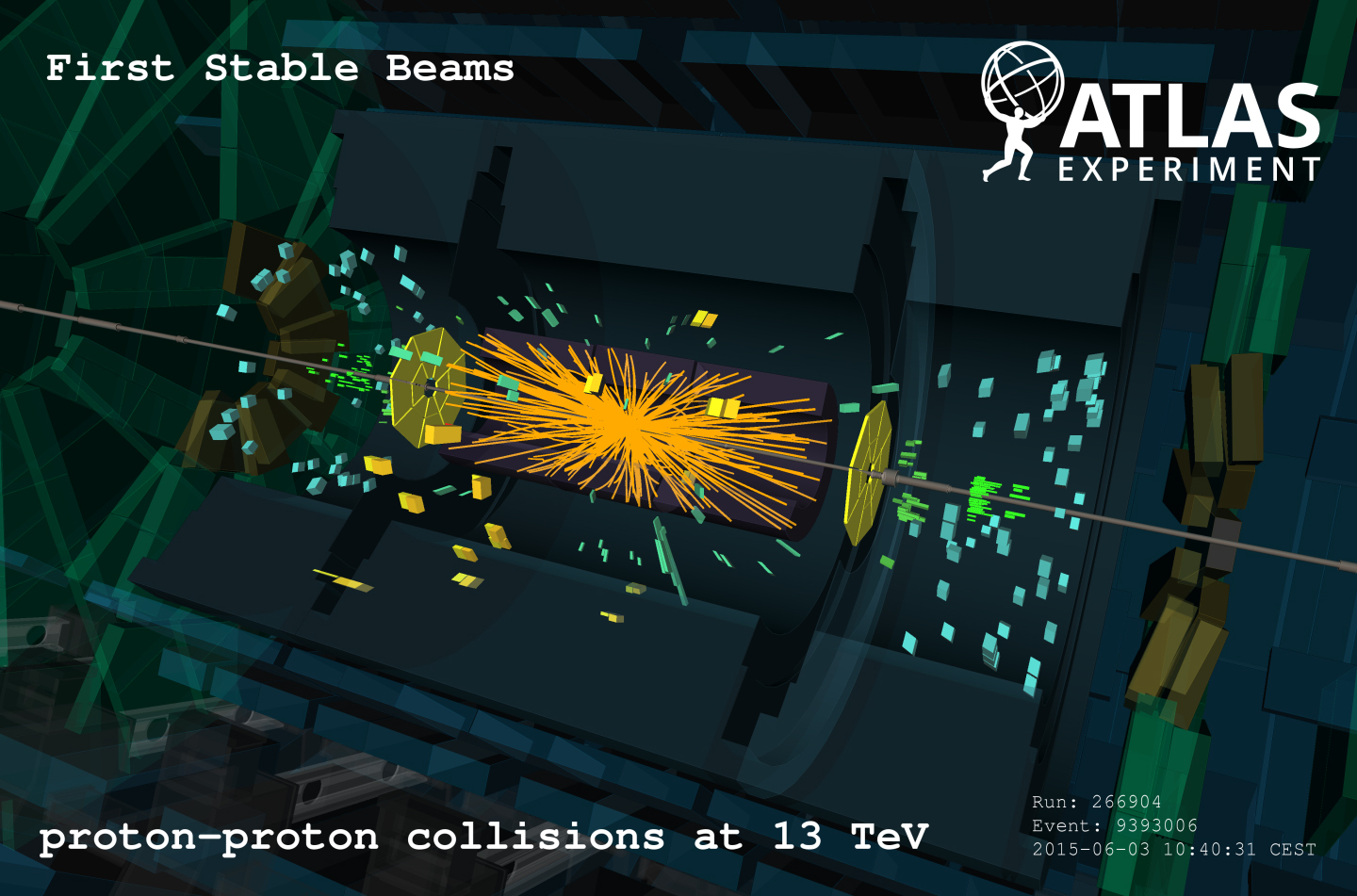This detailed digital illustration depicts a simulated view of a particle collision similar to those observed in the Large Hadron Collider's experiments. Central to the image is the dynamic representation of a proton-proton collision, rendered in vivid colors including orange, yellow, gray, green, blue, and dark green. It's a 3D rendering shown from a slightly overhead angle, capturing the essence of the high-energy event. In the top left corner, "First Stable Beams" is inscribed in white text, while the top right corner bears the label "Atlas Experiment." The bottom left corner of the image details "Proton-Proton Collisions at 13 TeV," and in the bottom right corner, specific experiment identifiers such as "Run 266904 Event 9393006 2015 June 3, 104031 CEST" are displayed. The overall composition effectively conveys the sophisticated and precise nature of the experiment conducted by the ATLAS collaboration.